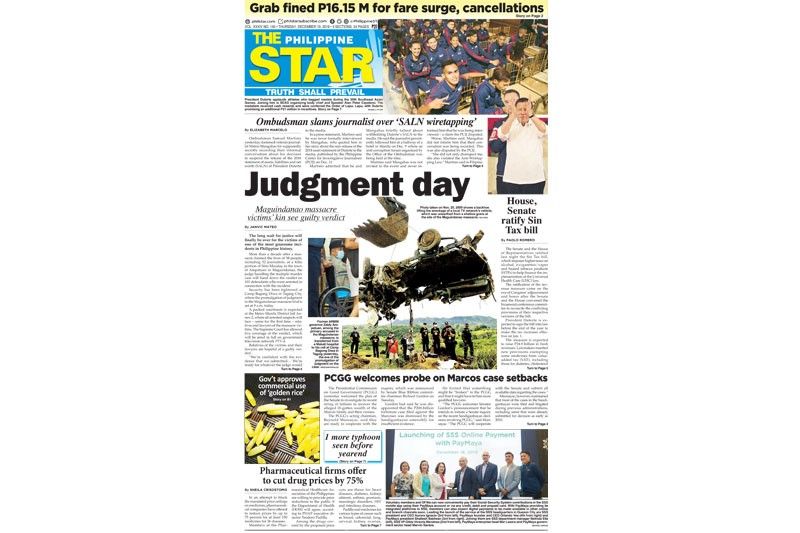This is an image of the front page of The Philippine Star newspaper. At the very top, a headline spanning from left to right reads, "Grab find P16.15M for fare search cancellations." 

Below this, the newspaper's nameplate prominently displays "THE" in yellow, followed by "PHILIPPINE" in white, capitalized but in a smaller font. The word "STAR" appears in even larger, bold capital letters, set against a blue background with yellow accents.

To the right, there is a photograph depicting several people sitting side by side. One individual in the front is making a peace sign.

Below the image, an article headline reads, "Ombudsman slams journalist over slain wire tapping." Adjacent to this, another article is titled, "Judgment Day."